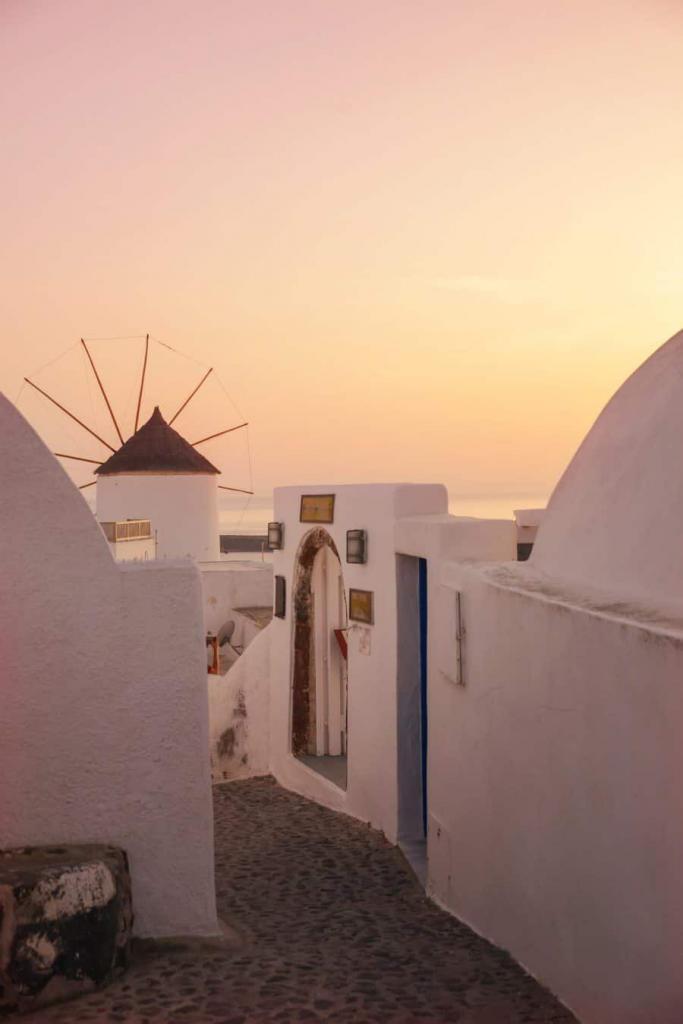In this color photograph, which is in portrait orientation, the foreground displays a picturesque, adobe-style courtyard of white stucco buildings, typical of Santorini, Greece. The top half of the image captures a serene peachy-orange, sunset sky, transitioning to an orangey-yellow hue towards the right, where the sun is likely setting.

Central to the composition, a narrow, dark pathway of brown pebbles leads inward, bordered by short white stucco walls. On the right, a partially visible dome-shaped roofed building cuts off the image's edge. This building features a doorway opening towards the center. Adjacent to this, further along the path, is an arch and a blue door.

On the left, another arched structure with a straight-edged wall in the center draws the viewer's eye. In the background, towards the horizon, a distinctive tower with a dark triangular roof stands out. Before this tower, a windmill with brown spokes adds character to the scene. Peeking through the gaps between these buildings, the ocean reflects the soft, warm hues of the sky, enhancing the overall tranquility of the image.